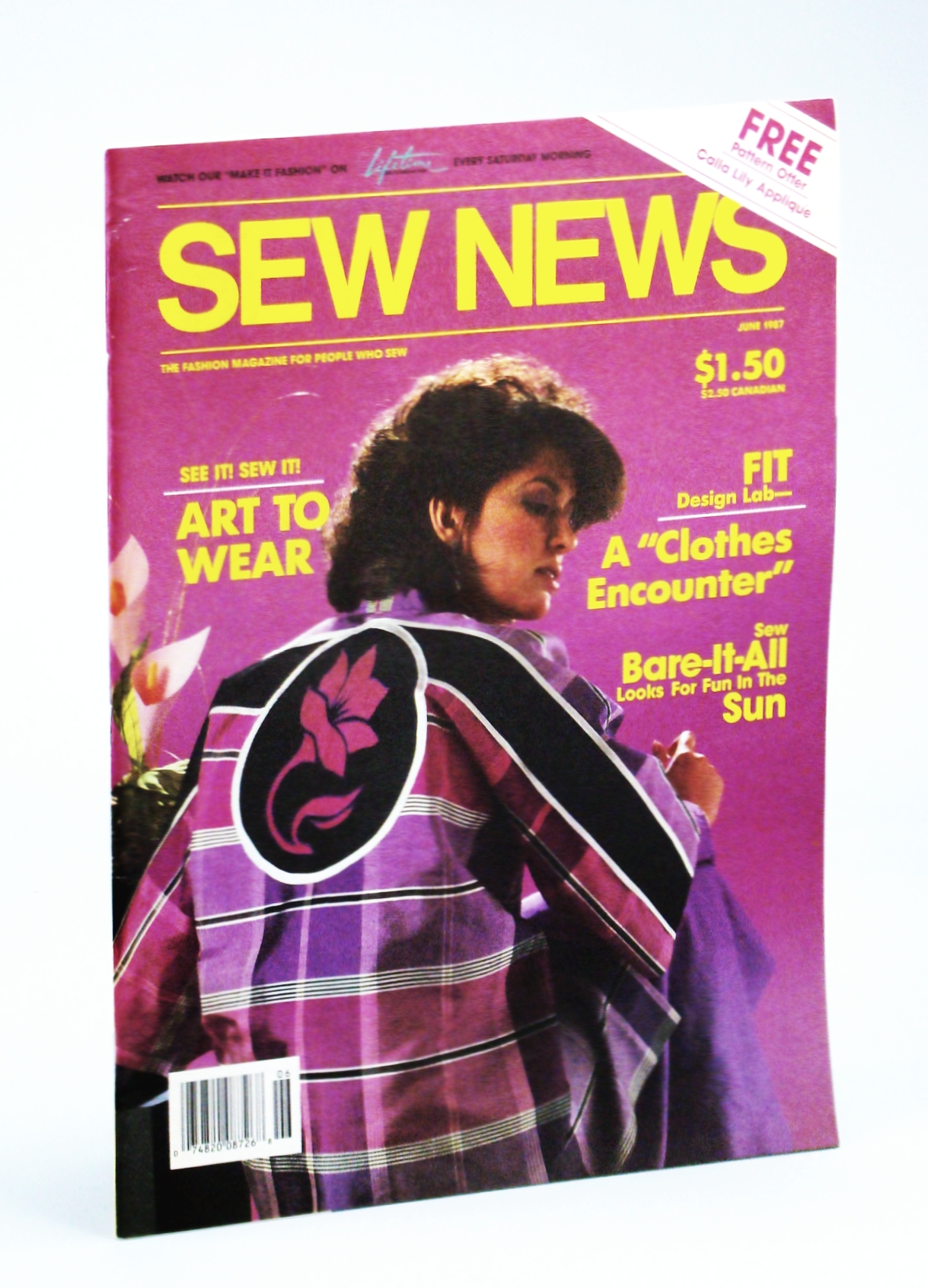The image captures the cover of a vintage magazine titled "Sew News," dating back to June 1987, a fashion magazine tailored for sewing enthusiasts. The cover is characterized by a vibrant palette of bright yellow text set against shades of pink and purple. Dominating the scene is a model with a quintessentially 80s curly hairstyle. She faces slightly over her right shoulder, offering a view primarily of her back. Her attire features a fuchsia purple, black, and white plaid top embellished with a distinctive oval patch on the back. This patch has a black background with a white border and a fuchsia flower at its center. The magazine also lists several headlines in bright yellow lettering, including "See It, Sew It, Art to Wear," "Fit Design Lab, A Clothes Encounter," and "Sew, Bear It All, Looks for Fun in the Sun." Additional details on the cover include a barcode in the lower left-hand corner and a notification in the top right-hand corner for a "Free Pattern Offer" featuring a Calla lily applique. The cover price of the magazine is marked at $1.50.